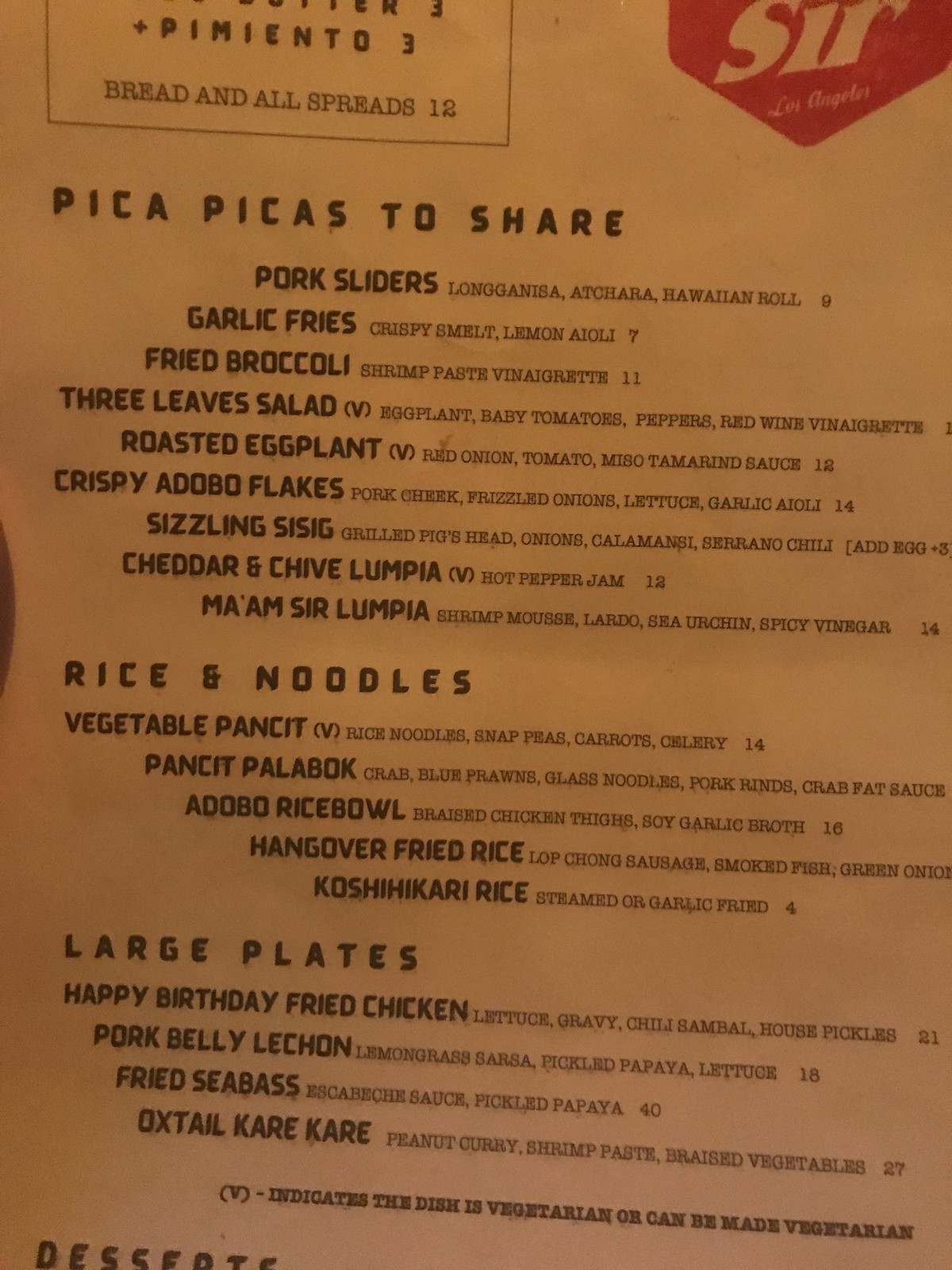**Menu for Sir SIR Los Angeles**

(The menu has a tan hue, which may be due to shadowing on a white background.)

**Appetizers**  
- Pimento 3  
- Bread and All Spreads 12  

**Picas to Share**  
- Pork Sliders  
- Longaniza  
- Octaria  

**Specialties**  
- Hawaiian Roll 9  
- Garlic Fries  
- Crispy Smelt with Lemon Aioli 7  
- Fried Broccoli with Shrimp Paste Vinaigrette 11  
- 3-Leaf Salad: Eggplant, Baby Tomatoes, Peppers, Red Wine Vinaigrette  
- Roasted Eggplant, Red Onion, Tomato, Miso, Tamarind Sauce 12  

**Signature Dishes**  
- Crispy Adobo Flakes: Pork Cheek, Frizzled Onions, Lettuce, Greek or Garlic Aioli 14  
- Sizzling Sisig: Grilled Pig's Head, Onions, Calamansi, Siriano Chili (Add Egg +3)  
- Cheddar and Chive Lumpia with Hot Pepper Jam 12  
- Ma'am Sir Lumpia: Shrimp Mousse, Lardo, Sea Urchin, Spicy Vinegar 14  

**Rice and Noodles**  
- Vegetable Pancit: Rice Noodles, Snap Peas, Carrots, Celery 14  
- Pancit Palabok: Crab, Blue Prawns, Glass Noodles, Pork Rinds, Crab Fat Sauce  
- Adobo Rice Bowl: Braised Chicken Thighs, Soy Garlic Broth 16  
- Hangover Fried Rice: Longsilog Sausage, Smoked Fish, Green Onion, Koshihikari Rice, Steamed or Garlic Fried 4  

**Large Plates**  
- Happy Birthday Fried Chicken: Lettuce, Gravy, Chili, Sambal, House Pickles 21  
- Pork Belly Lechon: Lemongrass Sarsa, Pickled Papaya, Lettuce 18  
- Fried Sea Bass with Escabeche Sauce and Pickled Papaya 40  
- Oxtail Kare-Kare: Peanut Curry, Shrimp Paste, Braised Vegetables 27  

*(V indicates dishes that are vegetarian or can be made vegetarian)*